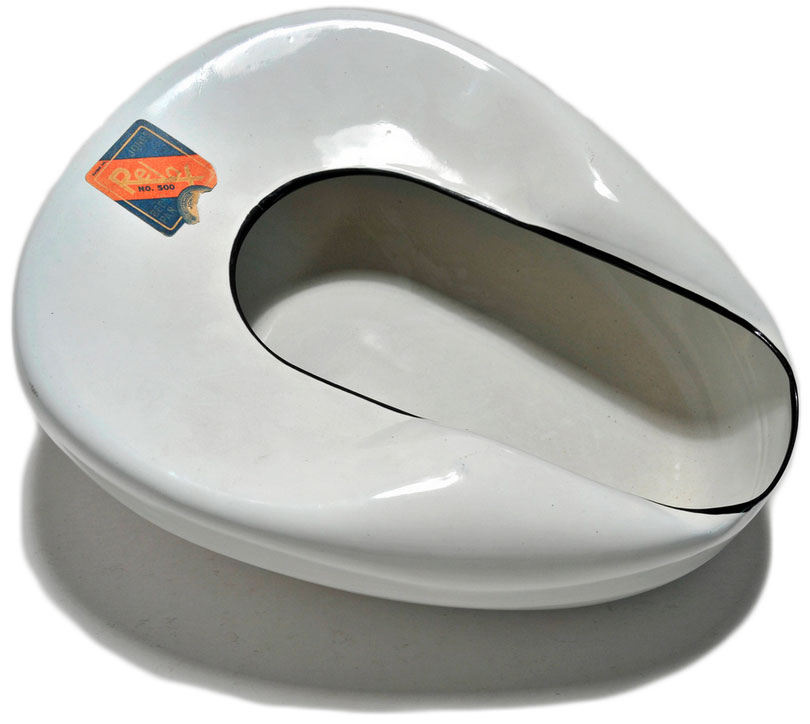The image showcases an enigmatic, museum-like piece of pottery or possibly an abstract art object. It is predominantly white and glossy, suggesting it may be porcelain, and features a dark rim around its inner edge. The design is oblong or oval, with a hollow center resembling a filled-out toilet bowl seat or potentially a bowl or ashtray. The object bears a sticker that reads "relax number 500," with the number hyphenated to "NL." The high gloss gives it a shiny, almost pristine appearance. Positioned alone on a white surface with a noticeable shadow, this polished item could serve as a container for various items or simply be a display piece. Its precise function remains unclear, adding to its mysterious allure.